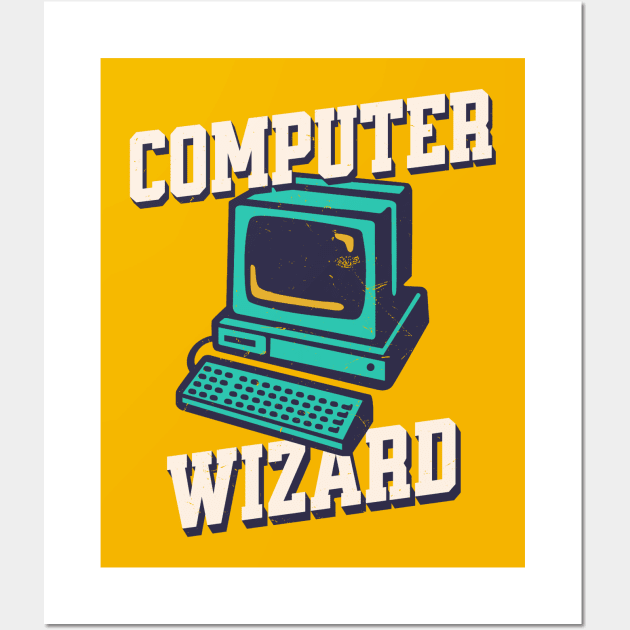This vibrant poster, set against a grayish white wall and framed with a white border, serves as an advertisement for a computer repair service named "Computer Wizard." Dominated by a golden yellow background, the center showcases a whimsical, cartoonish image of a vintage, turquoise-colored computer. The computer features an older, cathode ray tube monitor with a black screen, perched atop a similarly colored CPU unit. Notable details include a slot for a three-and-a-half-inch floppy disk and a circular black button, likely the power switch. The keyboard, positioned in front of the monitor, is depicted in aqua blue, obscuring parts of the text below it. Bold, all-capitalized white letters above and below the computer graphic spell out "COMPUTER" and "WIZARD," respectively, with the letters highlighted by a blue layer that imparts a 3D effect to the text. The nostalgic design suggests it might be an outdated advertisement from a time when floppy disks and cathode ray tube monitors were prevalent.